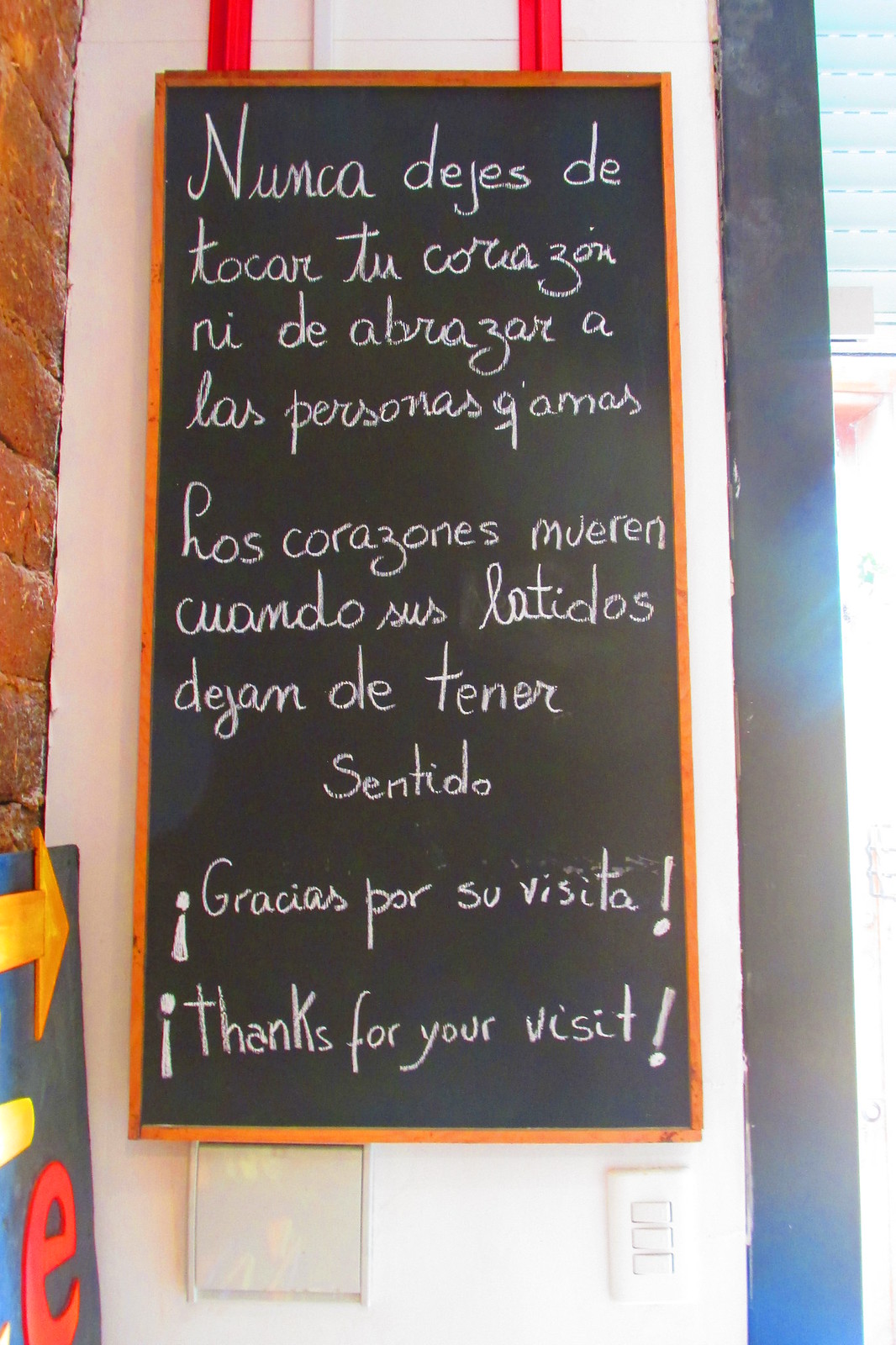The image depicts a chalkboard with a wooden frame, attached to a red brick wall adorned with a blue sign featuring a yellow arrow and a red "E". The chalkboard appears to be located in a restaurant, as suggested by the welcoming message written in Spanish, which says, "Nunca dejes de tocar tu corazón. Ri de abrazar a las personas jamás. Las corazones mueren cuando sus latidos dejan de tener sentido. Gracias por su visita." This translates to "Never stop touching your heart. Laugh at hugging people never. Hearts die when their beats stop making sense. Thanks for your visit." The text is written in a mix of regular and cursive handwriting. The scene is brightly illuminated by sunlight coming from the right side of the image, suggesting proximity to a window or door. Adjacent to the bottom of the chalkboard, there is a light switch panel with three knobs.